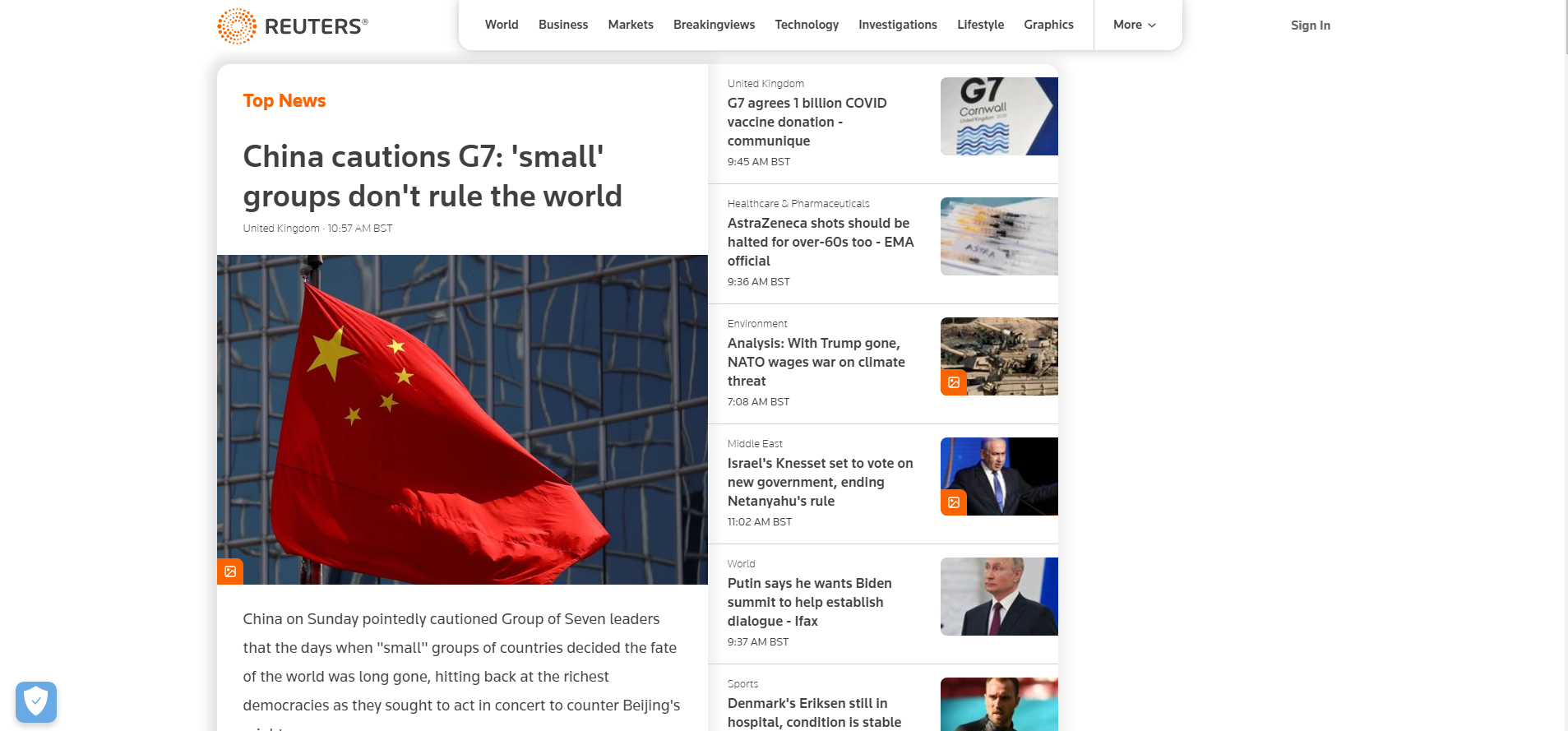This is a detailed screenshot from the Reuters website. At the top, "REUTERS" is displayed in bold, black, capital letters. A navigation menu is located to the right, featuring categories such as "World," "Business," "Markets," "Breakingviews," "Technology," "Investigations," "Lifestyle," "Graphics," and a "More" option with a drop-down menu. 

On the left side of the screenshot, there's the header "Top News." Below it, the story titled "China cautions G7: small groups don't rule the world" is mentioned, marked as "United Kingdom 10:57 a.m. BST." Accompanying this news is a photograph of the Chinese flag in front of a mirrored building. Beneath the photo, there's a partial excerpt stating, "China on Sunday pointedly cautioned Group of Seven leaders that the days when 'small' groups of countries decided the fate of the world was long gone, hitting back at the richest democracies as they sought to act in concert to counter Beijing's...". The text cuts off at this point.

Directly to the right, the next story titled "G7 agrees 1 billion COVID vaccine donation communique" is listed, marked "9:45 a.m. BST." The article is illustrated with a photograph of a "G7 Cornwall" sign, featuring a dark and light blue wavy design beneath it. 

To the right of that, another news piece is titled "AstraZeneca shot should be halted for over 60s too, EMA official," noted as "9:36 a.m. BST." This story is accompanied by an image of multiple syringes laid out on a white surface.

Further to the right, the "Environment" section features an article "Analysis: With Trump gone, NATO wages war on climate threat," dated "7:08 a.m. BST." The article includes a photo of an arid landscape.

To the far right, a piece in the "Middle East" category titled "Israel's Knesset set to vote on new government ending Netanyahu's rule" is marked at "11:02 a.m. BST." The article's image depicts a middle-aged man, seemingly wearing a dark suit, white collared shirt, and blue necktie, looking downward.

Below this, under the "World" category, the headline "Putin says he wants Biden summit to help establish dialogue, IFAX" is dated "9:37 a.m. BST." It's accompanied by a photograph of Vladimir Putin, who appears to be looking leftward with raised eyebrows, dressed in a dark suit jacket, white collared shirt, and red necktie.

Finally, in the "Sports" section, the headline "Denmark's Eriksen still in hospital, condition is stable" is given without a timestamp. To the right, there's an image of a white man, possibly a soccer player, with furrowed brows looking to the left.